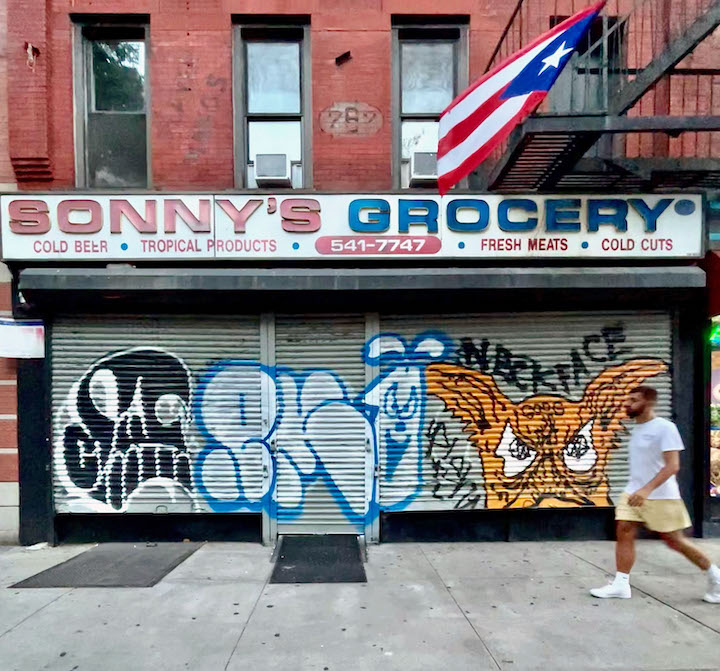The photograph captures a storefront on a relatively warm, cloudy day. The upper portion of the building is an older-style brick structure with a black metal balcony and three clear glass windows with gray frames. Two of these windows have visible air conditioners. The lower portion features closed roll-up doors covered in graffiti, including a black skull, a little gremlin face, a black caterpillar, and an orange creature with big ears. Above the store, a white banner displays in red and blue text: "Sunnies Grocery" followed by "Cold Beer, Tropical Products, Fresh Meats, and Cold Cuts," along with a phone number prominently featured in a red pill shape: "541-7747." A man with short black hair and a black beard is walking on the sidewalk in front of the store, dressed in a white short-sleeved shirt, cream-colored shorts, white socks, and white shoes. The sidewalk is composed of large gray square tiles. A red, white, and blue flag with three red stripes, two white stripes, a blue portion, and one star is visible at the top of the shop.